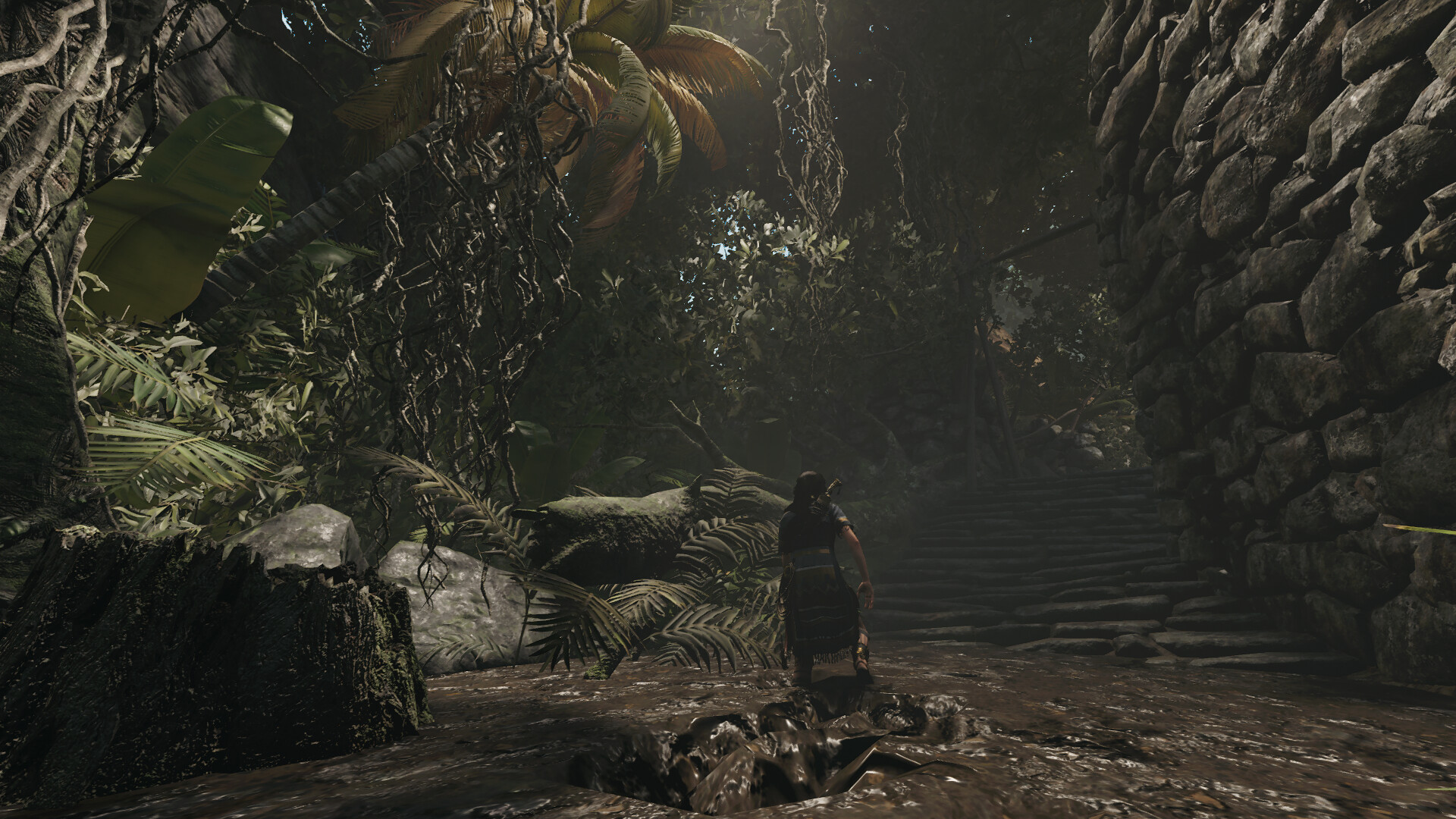This image appears to be from a video game or a computer-generated scene, depicting a muddy, swamp-like environment. The ground is saturated with mud, which seems to ripple and flow like liquid. In the foreground, a person with long black hair is dressed in a fabric skirt and equipped with various weapons and sturdy boots. They are walking towards a series of stone steps emerging from the mud.

To the right of the scene, there is a massive stone wall composed of giant stones, lending an ancient and imposing feel to the setting. On the left side, the environment is lush with dense foliage, including gray rocks protruding from the mud. Among the greenery, a palm tree stands out with scraggly, brown vines hanging from it, along with an assortment of tree trunks and large, broad-leaved plants. 

Further ahead, more palm leaves can be seen, blending into the jungle foliage in the distance. The overall lighting of the scene is dim, with minimal natural light filtering through, adding to the dark and mysterious atmosphere of the swamp.